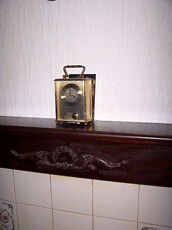In the image, a singular object rests delicately on a brown ledge with a gray logo on its front. This object resembles a square lantern with yellow outer edges and a gray handle on top. Inside the lantern, there is a very small clock featuring a circular black outer frame and a white inner frame. The ledge is positioned against a backdrop comprised of white and light gray walls, while below the ledge, the wall transitions into a square white tiled design.